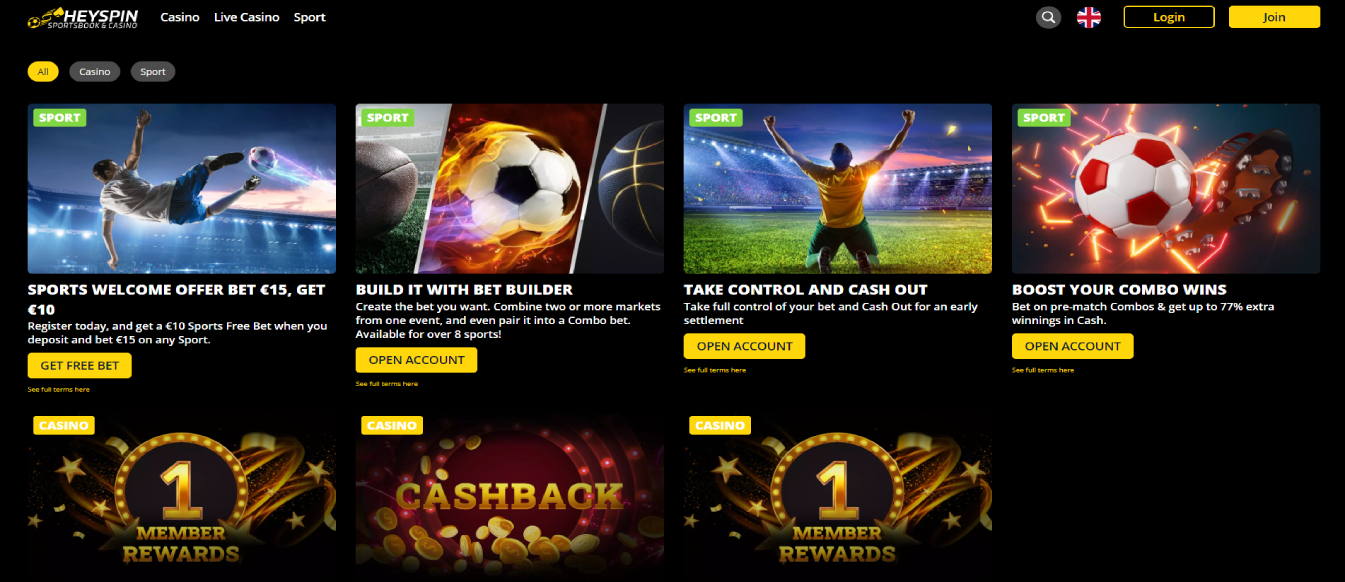This image is a detailed screenshot of a website named HeySpin, characterized by a predominantly black background giving it a sleek and dark aesthetic. In the top left corner, the website’s logo is displayed, featuring an image that resembles a soccer ball in motion beside the word "HEYSPIN" written in bold, capital letters. Adjacent to the logo is a tagline or subtext, though it is too small to be legible.

To the right of the logo, a navigation menu lays out options such as "Casino," "Live Casino," and "Sport." Further to the right in the top corner, you'll find a search icon housed in a gray circle, a button displaying the British flag, presumably for language selection, and two prominent buttons. The first is a "Log In" button, outlined in yellow with the text in yellow on a black background, and the second is a "Join" button featuring black text on a solid yellow background, all with rounded corners.

Below the navigation bar, there are three filter buttons labeled "All," "Casino," and "Sports." "All" is currently selected, indicated by its yellow background and black text, while the others have a gray background with white text.

Further below, the content area showcases seven tiles arranged in two rows – four tiles in the first row and three in the second. Each tile includes a thumbnail image in a 3:2 aspect ratio, along with labels indicating either "Sports" or "Casino." 

The first tile on the top left corner is labeled "Sports" in a green rectangle and illustrates a person kicking a soccer ball. Below the image, the text promotes the “Sports Welcome Offer” with a message: "Bet 15 euros, get 10 euros. Register today and get a 410 sports free bet when you deposit," followed by a call-to-action in a yellow button with black capital letters reading "GET FREE BET."

The subsequent tiles maintain a similar format, each containing a unique thumbnail with either a sports theme or casino-related imagery. Notable is the second row, where two tiles feature a repeated design: a golden-framed graphic labeled "Member Awards," suggesting a recurring game or event within the casino category, denoted by white text "Casino" within a yellow rectangle.

Each element contributes to a structured and visually appealing layout designed to engage the user with various promotional offers and navigational ease.